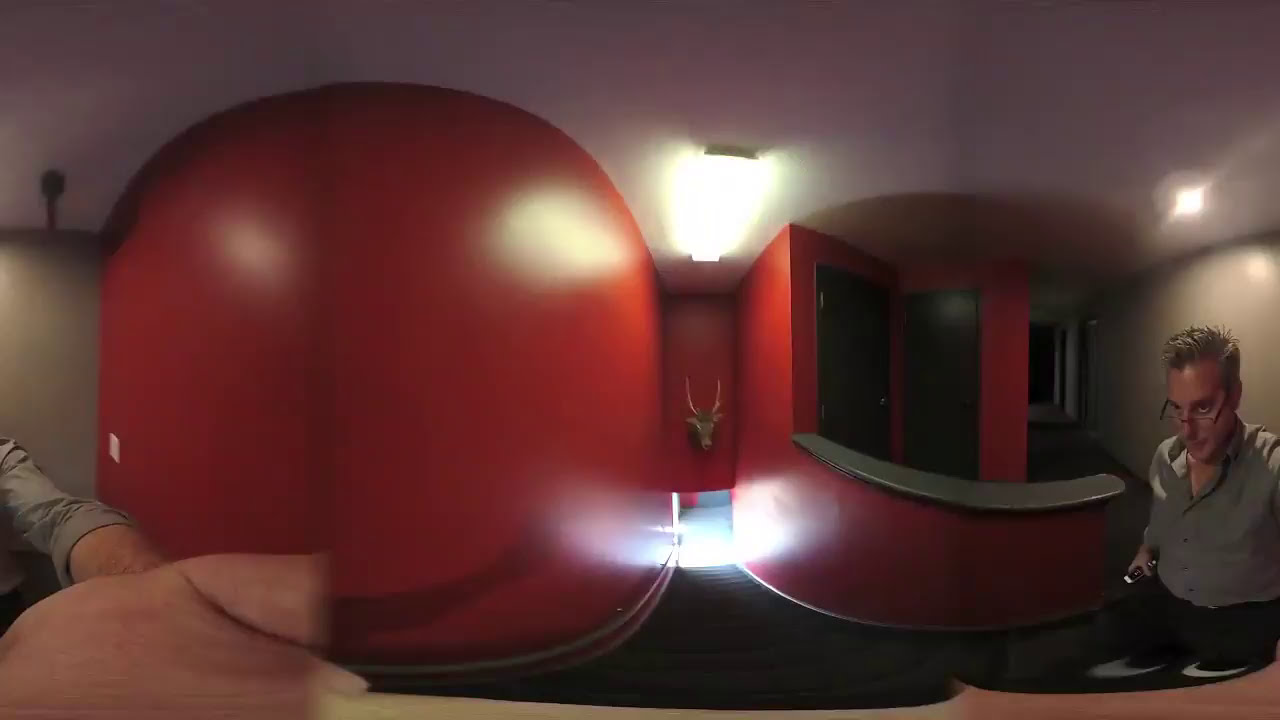The image appears distorted due to the use of a fisheye lens, giving a unique, bulging effect to the scenery. At the center of the image is a man wearing glasses and a long-sleeved gray shirt, black pants, and white shoes. His short, spiky hair is a mix of gray and black. He seems to be taking a selfie using a selfie stick or possibly holding a flashlight. The distortion affects his pose, making it seem like his arm, which extends outwards, reappears on the opposite side of the image.

The setting seems to be the interior of a building that could either be a hotel or possibly an office space. The ceiling is white and slightly darkened, with red walls dominating the scene. The corridor features multiple rooms with gray doors. A notable feature is the head of a moose mounted on the wall, adding a rustic touch to the decor.

On the left side of the image, there is a round bulging red section that resembles an over-sized cartoonish face with what appear to be eyes formed by white round dots and a darker red curved shadow suggesting a mouth. The image also includes a blurred hand stretching across the front, contributing to the surreal and distorted ambiance created by the fisheye lens.